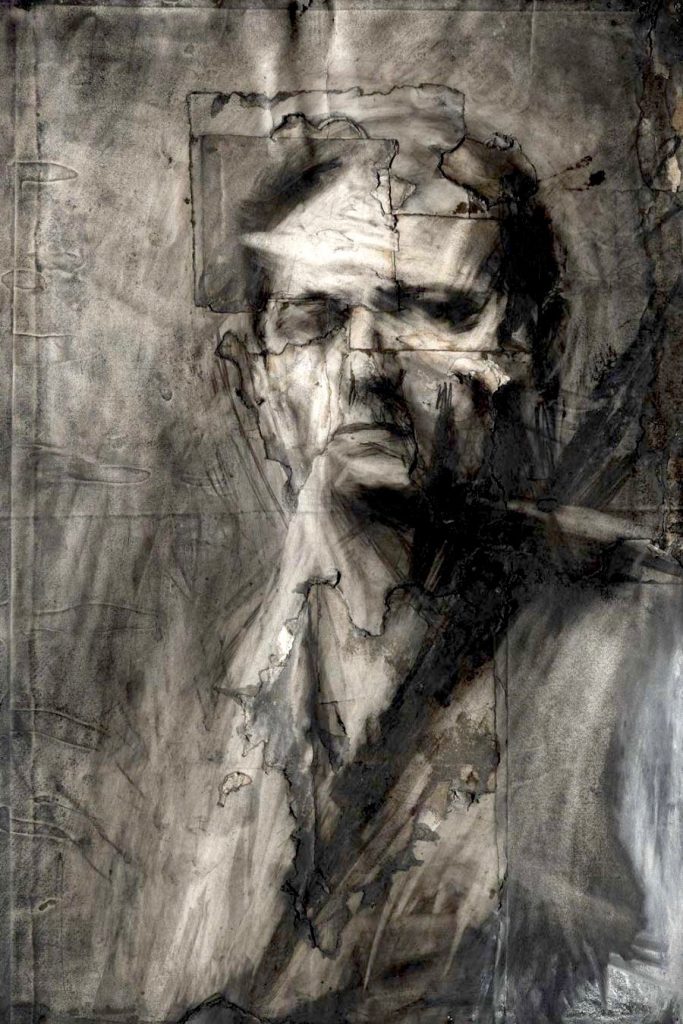This is an abstract black-and-white drawing of an older man with partially bald black hair and a receding hairline. The background is a textured mix of black, white, and gray with an almost antique, yellowy-gray tinge, possibly created using paintbrush strokes. The man's face is portrayed with a stark transition from a nearly silhouetted form at the bottom to a more detailed and visible face above. His expression is solemn with closed eyes, a prominent nose, and straight lips. A scar is noticeable beneath his left eye. He appears to be wearing a light-colored or white shirt with a V-neck, and a diagonal black strap crosses his chest, likely from a bag. The abstract nature of the drawing makes the outlines of his body indistinct and focuses more on piecing together his facial features with an intentional, perhaps taped, artistic effect that adds depth and interest.